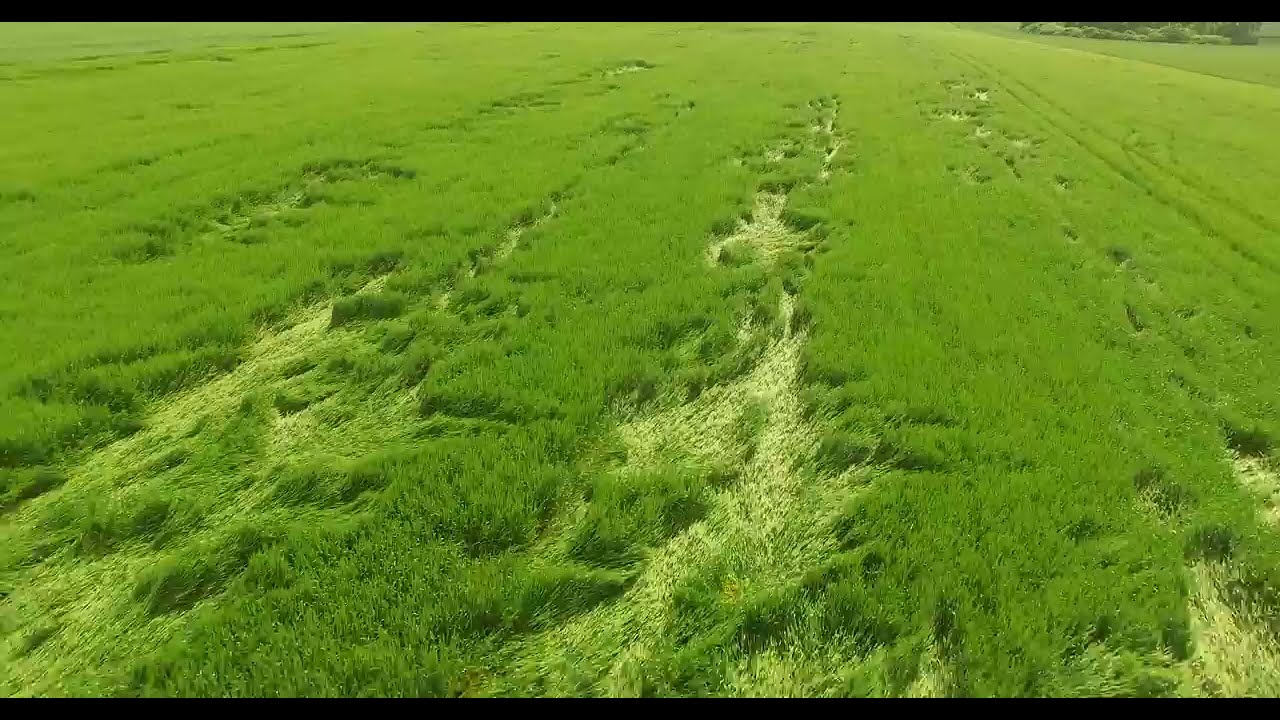The image is a color photograph capturing a large, lush field of tall, green grass. The grass appears very dense and verdant, with patches where the grass seems flattened, likely due to animal activity or maybe varying grass types. These flattened areas display shorter, lighter green, almost white-tinted grass, suggesting different growth stages or species. In the top right corner, you can spot a small section of green leaves from distant trees or bushes. The photo is framed in a letterbox format, with narrow black rectangles at the top and bottom, and it appears to be taken on a sunny day. There are no people, buildings, or other structures visible, emphasizing the expansive, uninterrupted green field.